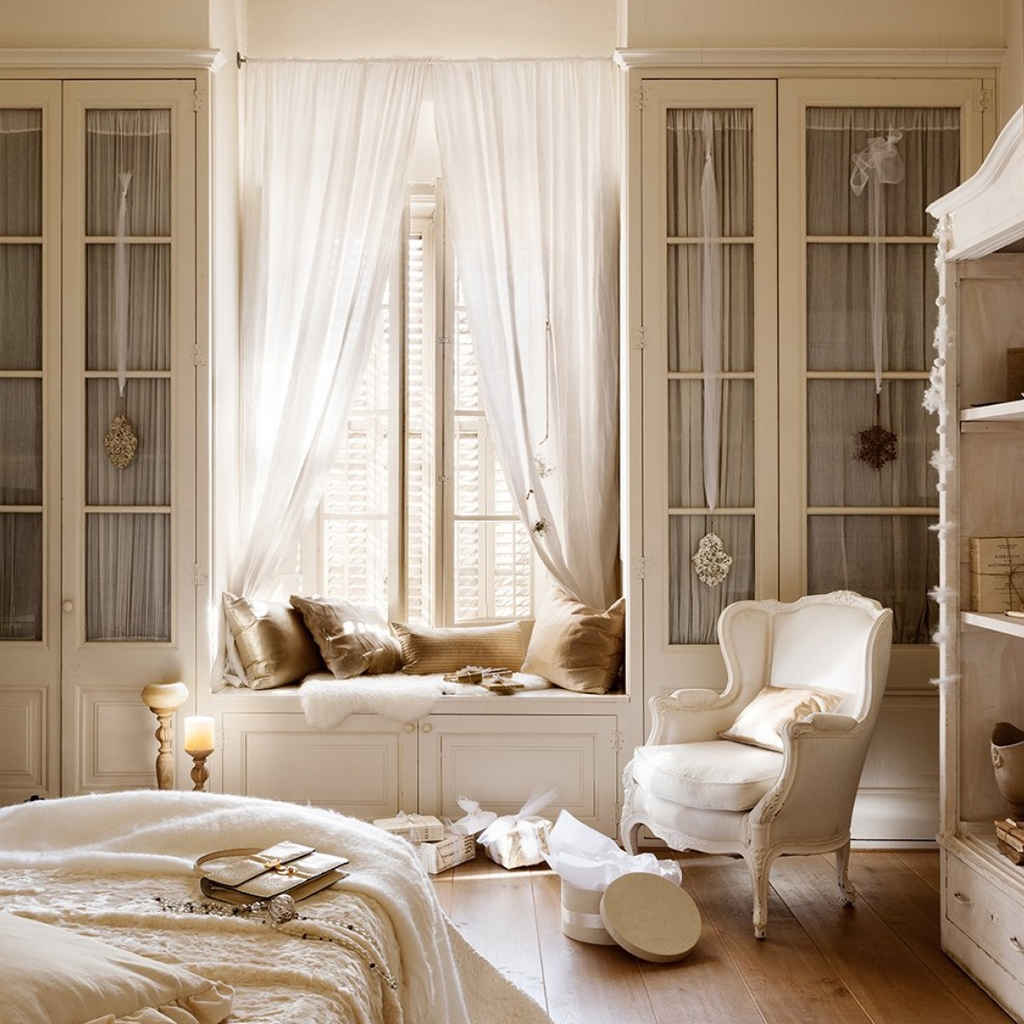This detailed image captures a very fancy and cozy room, dominated by beige and gold hues. Central to the room is a large window adorned with white silk drapes, which are tied back to allow light to stream in, creating a warm, yellowish ambiance. The window features a seating area embellished with plush golden pillows, perfectly poised for city views.

On either side of the window are two cupboards, each with double doors and decorative gold symbols hanging from white sheer ribbons. These cupboards are framed by gray curtains. In front of the window, there is an elegantly cozy white armchair, positioned beside a round box with white wrapping paper spilling out, as if someone was recently opening presents. Alongside this box are three other gold-wrapped presents.

A beige bed with white and gold-hued sheets is visible in the foreground, further emphasizing the room's lavish feel. A gold handbag rests on the bed, adding a touch of luxury. The wooden floor is a rich brown, complementing the room's overall decor. 

To the right of the room, there's a white bookshelf with an arched top and a drawer at the bottom, housing various books and vases. Tall candlesticks stand on the floor, contributing to the room's opulent atmosphere. The light flooding through the open window highlights the meticulous arrangement and sophisticated finish of this charming space.